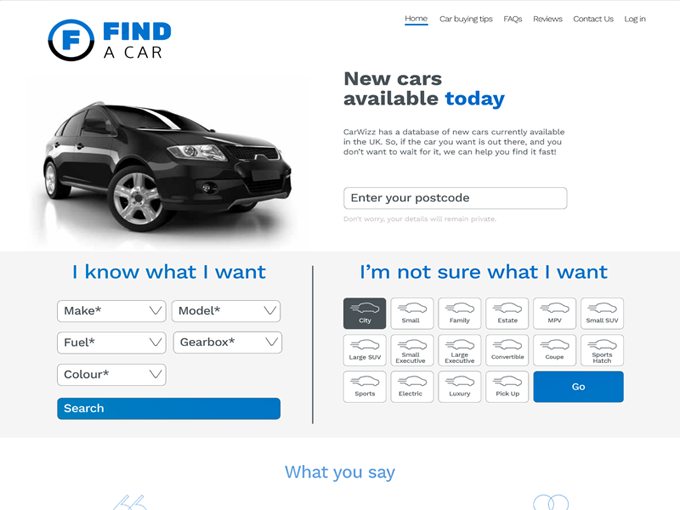The image depicts a sleek car website designed for user convenience and easy navigation. At the top left corner, prominently featured are the words "Find a Car," with "Find" highlighted in blue and "a Car" in black, suggesting a focus on searching for vehicles. Adjacent to this text, a logo is visible, consisting of a circle bisected into blue (top half) and black (bottom half), containing a blue "F" over a white background.

On the top right, a navigation bar provides links for "Login," "Contact Us," "Reviews," "FAQs," "Car Buying Tips," and "Home," with "Home" distinctively underlined in blue to indicate the current page.

Dominating the center-left of the image is a striking picture of a black SUV, emphasizing the type of vehicles available on the site. To its right, the text "New Cars Available Today" is displayed, with "Today" standing out in blue, drawing attention to the immediacy of the offers.

Below this, a rectangular search box invites users to "Enter Your Postcode," encouraging localized car searches. In the bottom left section, there is a feature titled "I Know What I Want," accompanied by five dropdown menus labeled "Make," "Fuel," "Color," "Model," and "Gearbox," enabling users to tailor their search precisely according to their preferences.